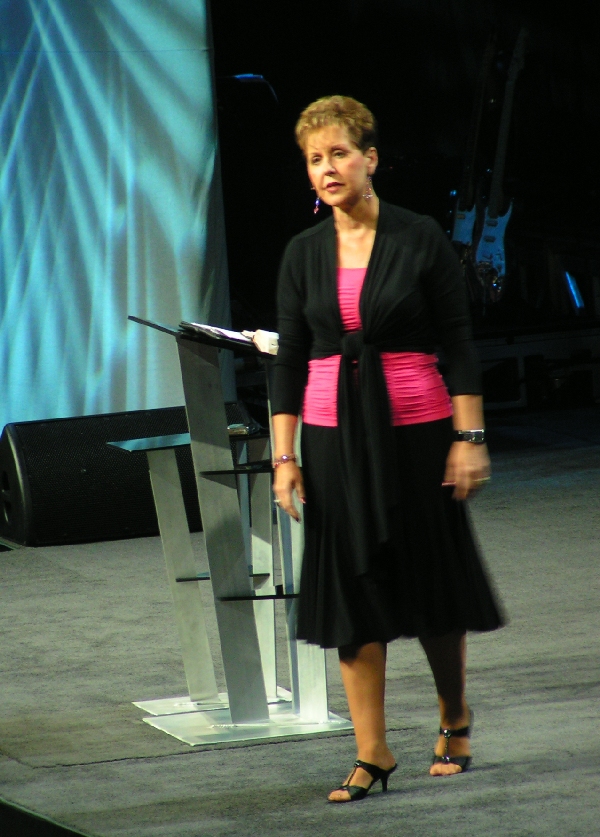The image showcases a woman standing on stage, positioned slightly to the left in front of a sleek silver podium. She has light brown, short curly hair and is adorned with long silver earrings. Her attire consists of a stylish black dress with a distinctive pink band around the waist and a pink shirt beneath it. On her left wrist, she wears a wristwatch, and on her right, a bracelet. Her feet are clad in elegant black high heel sandals. The background features a vertical rectangular screen displaying some graphics and is framed by light and darker blue curtains, suggesting a formal setting, possibly for a speaking engagement. Additional elements in the background include stereos and guitars towards the right, adding a musical ambiance to the scene. The stage floor is covered with gray carpet. The overall atmosphere is professional and organized, with the woman appearing as the focal point of the photograph.